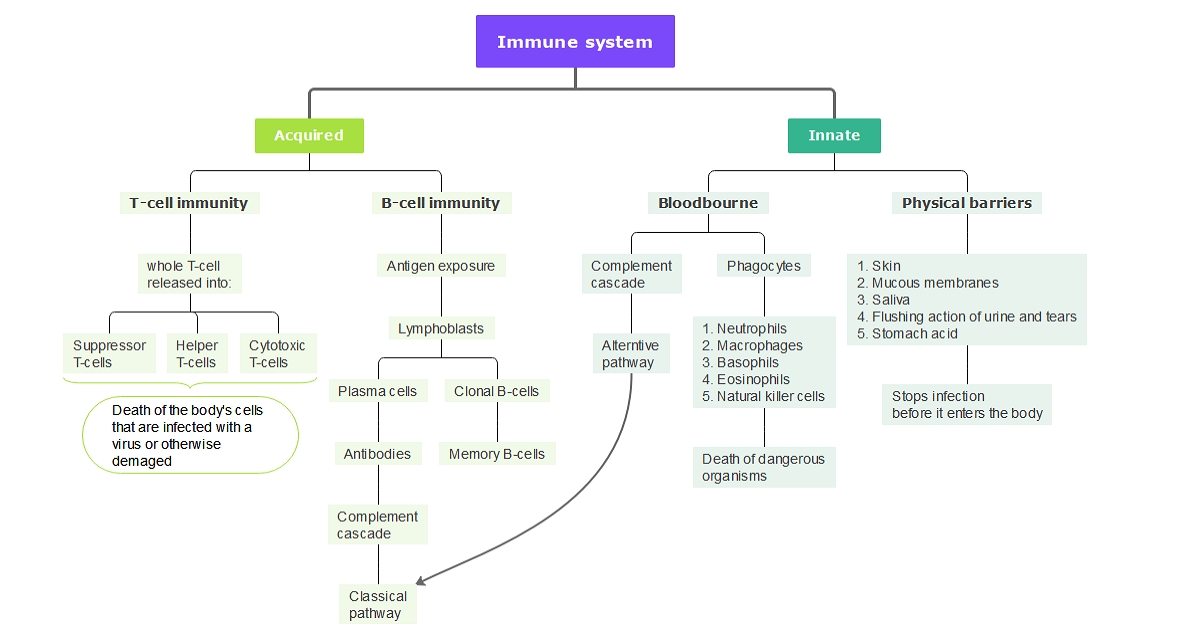The image is a detailed flowchart representing scientific information about the immune system, resembling a family tree with branching lines and text labels. At the top, a prominent purple rectangle with white text reads "Immune System." From this central node, two primary branches extend downwards: one in a shade of green labeled "Acquired" and the other in a different shade of green labeled "Innate."

Descending from the "Acquired" branch are further subdivisions indicating "T-cell immunity" and "B-cell immunity." Additional labels under this branch include "Suppressor T-cells," "Helper T-cells," "Cytotoxic T-cells," and "Antigen exposures." 

The "Innate" branch bifurcates into categories such as "Blood-borne" and "Physical barriers." A notable detail under "Blood-borne" includes an arrow pointing from "Alternative Pathway" to "Classical Pathway." Under "Physical barriers," there is a comprehensive list in a box that includes:

1. Skin
2. Mucous membranes
3. Saliva
4. Flushing action of urine and tears
5. Stomach acid

There are also labels for "Plasma cells," "Antibodies," and "Complement cascade." At the bottom left corner, a small bubble emphasizes the endpoint of certain immune responses, stating: "Death of the body cells that are infected with a virus or otherwise damaged."

Overall, this gray flowchart with interconnecting boxes vividly illustrates the intricate mechanisms and components of the immune system, distinguishing between its acquired and innate branches.